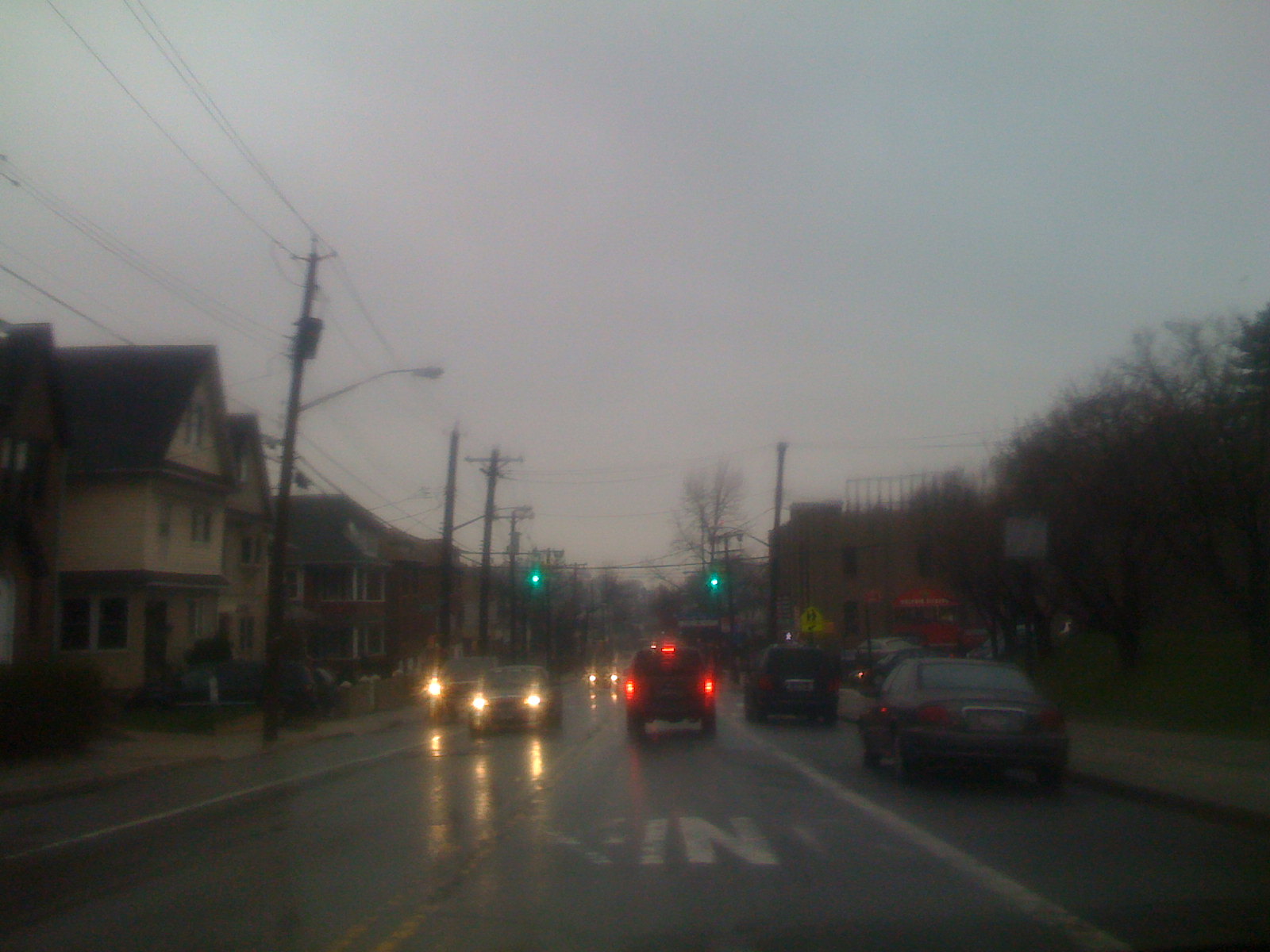The image features a two-lane road marked by a double yellow line running down the center and white lines on both the left and right edges. Multiple cars are visible: a brown car and a black car are traveling towards the center of the image, while other cars on the left side are heading towards the bottom right. A green traffic light is present in the middle of the scene. 

On the left side of the road, there's a cream-colored house with a black roof and a black car parked in front of it. In the background, power lines and cables stretch across the road. A yellow street sign is visible on the right side in the foreground, and additional houses can be seen further down the road.

Trees line the right side of the image, providing a green backdrop. At the bottom of the image, white text with some letters scratched off is visible on the right lane, with the discernible letters forming the word "IN".